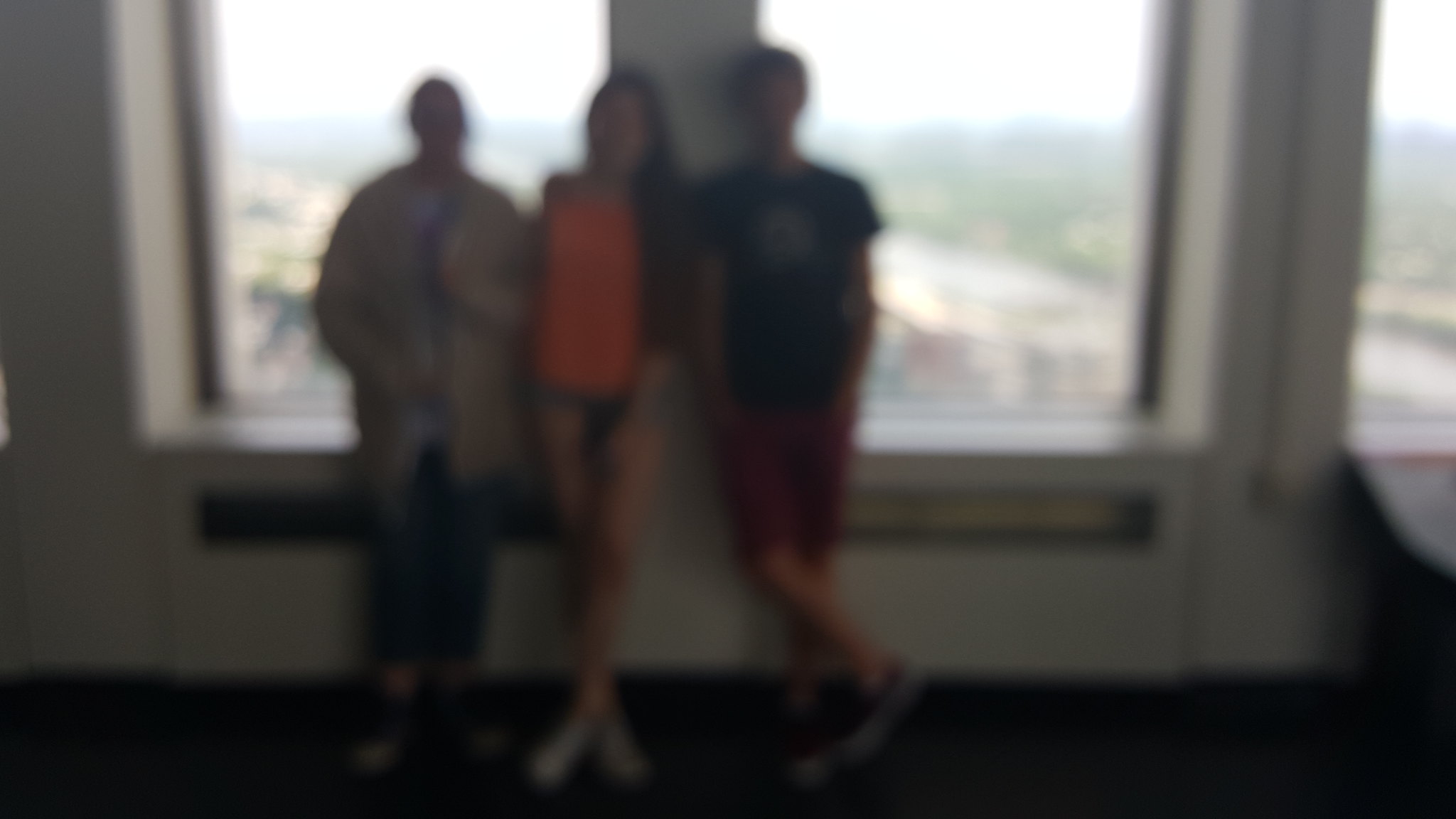The image depicts a blurry group photo of three people standing against a wall with large windows. The central figure is a girl with almost waist-length hair, dressed in an orange top, short denim shorts, and white shoes. To her right is a boy wearing a dark blue t-shirt with a white graphic in the middle, red shorts, and blue and white shoes, casually leaning against the wall with his hands in his pockets. On her left stands another boy in a blue shirt with a tan long-sleeve button-up shirt over it and blue jeans, sporting very short hair or possibly bald. The scene is set inside a building with large windows in the background, through which a vast cityscape is visible, suggesting they are at the top of a building.